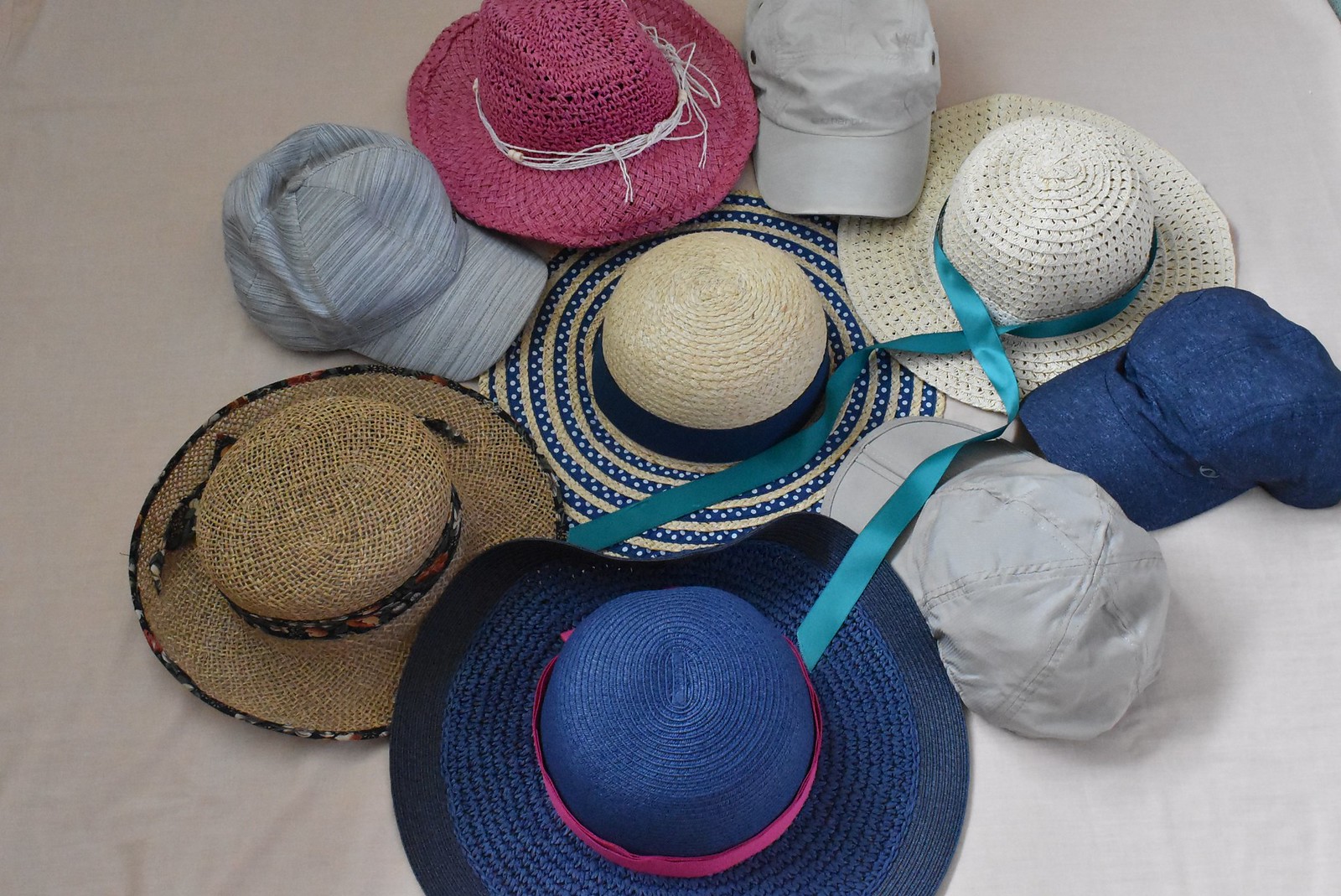This overhead photograph displays nine women's hats arranged on a soft, white cloth surface in a circular pattern, centering around one prominent hat. The central hat is a wicker straw-looking sunhat with a flat, wide brim, featuring alternating tan and blue stripes and adorned with a blue ribbon tied around its base. Moving clockwise from the top, the first hat is a pink straw hat with a white string around it. Next, there's a light blue cap with its bill facing downward, followed by another tan sunhat similar to the central one, featuring a long blue ribbon that extends to the left. Further down, a dark blue cap with a straightforward design and no logos is positioned facing the central hat. Below the central hat is its dark blue version, distinguished by a pink ribbon. Continuing upwards, there is a straw-colored sunhat with a floral-patterned trim around its brim and a matching floral ribbon around its base. Lastly, the collection ends with a simpler gray and dark gray striped cap. Most hats are designed for sunshade, though some are simple caps without logos, intended for women.